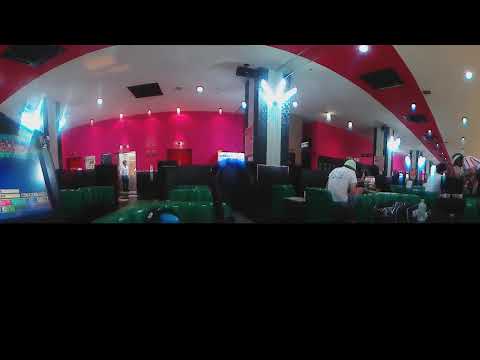The image captures an indoor scene of a dimly lit cafe or restaurant with a unique 360-degree perspective causing some visual distortion. The back wall of the establishment is painted red and features white lights that illuminate the area. The ceiling, predominantly white, also shows some red hues due to the lighting. Green cushioned booths occupy the foreground. The left side of the image shows a blue wall adorned with various signs. A customer, seated front and center, wears a white t-shirt and a blue or light green stocking hat. Additionally, a person is bent over a table on the right, possibly a server, also in a white shirt. The image is framed by thick black rectangles on the top and bottom, adding to the unusual visual characteristics.